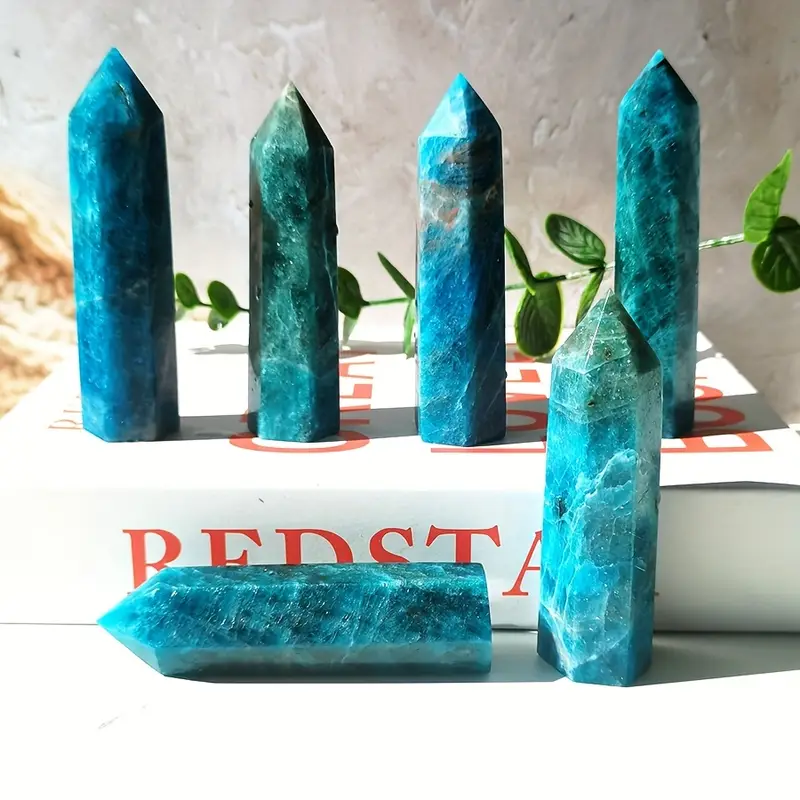This photograph captures a vivid arrangement of six bright blue or turquoise crystals, meticulously carved into tapered, octagon-like shapes reminiscent of pencils or candles. Each crystal is finely detailed, with some featuring marbled streaks of white and splashes of pink, adding to their visual complexity. They stand or rest atop a prominent white book adorned with red lettering, though the specific text is obscured. This book sits on a white cardboard box, serving as the base for the display. 

In the background, a textured stone wall, subtly marbled and featuring slight orange accents on the left, provides a rustic backdrop. Adding a touch of nature, a vine with alternating circular green leaves sprawls across the scene. The well-lit setting enhances the rich colors and intricate details of the crystals, making the image both vibrant and captivating. The overall composition is square-shaped, carefully blending natural elements with an artistic arrangement of the carved minerals.